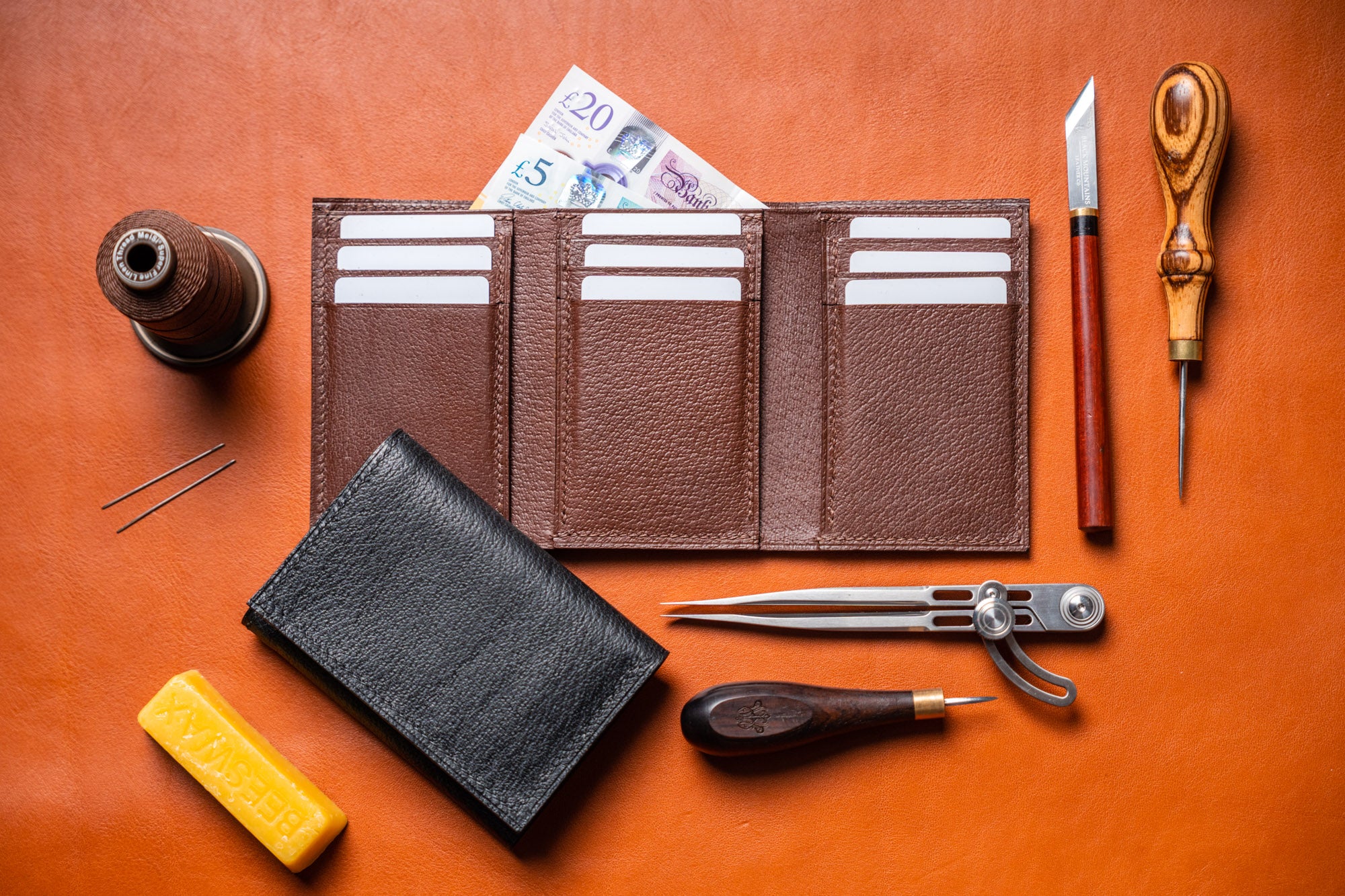The image is set on an orange background and features a detailed arrangement of items related to leather crafting. At the center, a brown leather wallet lies open, revealing its three sections, each holding three slots, with British pound notes peeking out. Below this wallet, towards the left, a closed black leather wallet rests, partially underneath the brown one. To the left side of the image, there's a yellow bar of beeswax. Above it, a spool of brown thread is situated. The top right area of the image includes a leather cutting knife with a red handle, a screwdriver with a wooden handle, and a sharp pick that resembles a large needle. Scattered around the wallets are various leather crafting tools such as an X-Acto knife, tweezers, a hole punch, a silver protractor, and two bobby pins. The entire setup suggests a workspace where wallets are crafted and repaired.